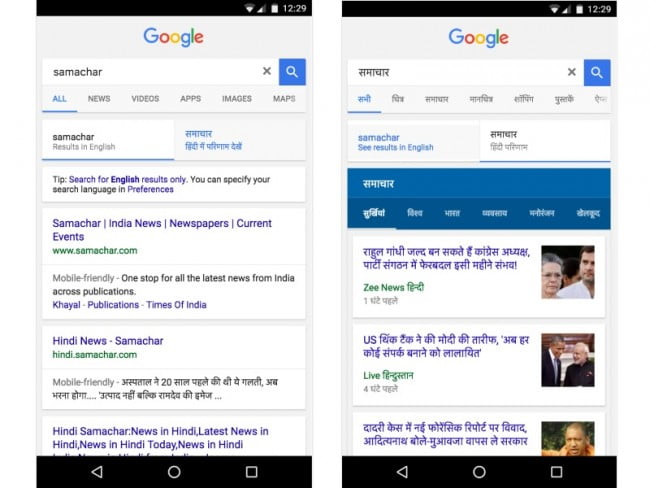The image showcases two screenshots side by side, depicting Google search results for the term "Samachar." Both screenshots are from an Android device, as evidenced by the interface design.

**Left Screenshot:**
- The screen displays the Google search bar at the top, complete with the Google logo.
- Below the search bar, the search term entered is "Samachar" in English characters (S-A-M-A-C-H-A-R).
- The active tab is "All," highlighted in blue, indicating a general search.
- Underneath the search bar, a white box prominently displays "Samachar" in bold, with the notation "results in English" in gray beneath it.
- To the right of this text, options in Arabic script are visible.
- A notification box just below suggests users can specify search languages and preferences, and it reads, "Tips, search for English results only."
- The search results listed include:
  1. "Samachar India News"
  2. "Hindi News Samachar"
  3. "Hindi Samachar News in Hindi"

**Right Screenshot:**
- This screenshot reflects a different tab selection from the previous one, switching from "results in English" to results in another language (possibly Hindi or Farsi).
- The new tab is highlighted in blue, while the English results are no longer selected.
- The search results are now presented in a non-English script.
- Three relevant websites are displayed, each accompanied by an image:
  1. "Z News" with a photo of a man and a woman.
  2. A website featuring an image of Barack Obama with another man.
  3. An entry showing a monk dressed in an orange robe.

This depiction provides a clear comparison between English and non-English search results for the term "Samachar" on Google, demonstrating how language selection influences the presentation of search outcomes.